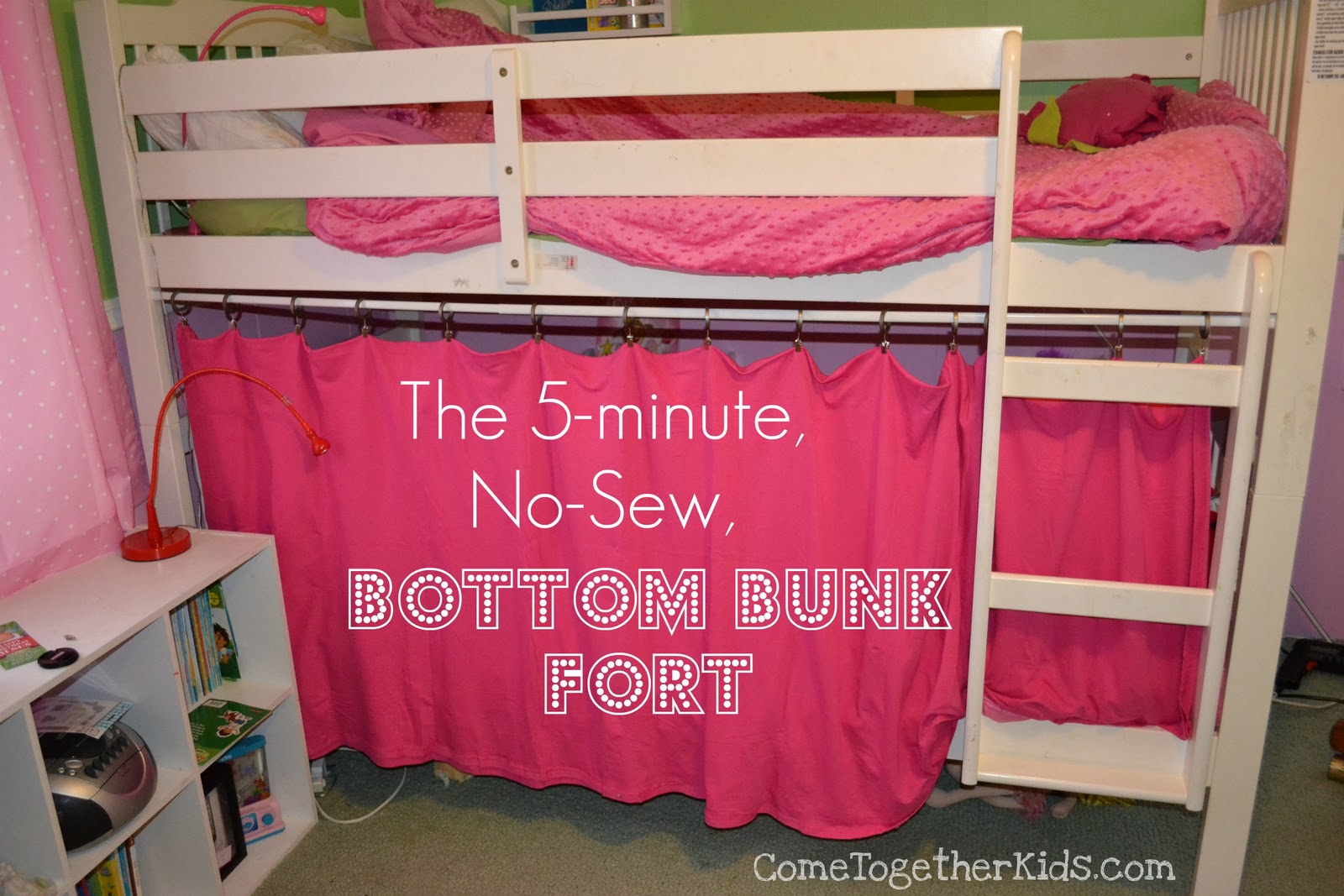This photograph captures a vibrant children's bedroom featuring a white wooden bunk bed. The top bunk is adorned with pink bedding and is accessed by a white ladder. The bottom bunk is not a bed but instead converted into a play area, concealed by a pink curtain. Superimposed on this curtain in white text are the words "The 5-minute no-sew bottom bunk fort." Adjacent to the bunk bed on the left, there is a white, four-compartment bookshelf filled with kids' books and an old CD player. To the right of the image, the text "cometogetherkids.com" is visible in white against the pink curtain. The bedroom's walls are painted in contrasting shades of dark green and purple, and a red lamp can be seen within the space, adding to the room's colorful decor. Another pink curtain, possibly for a window, is also visible on the left side of the photo.